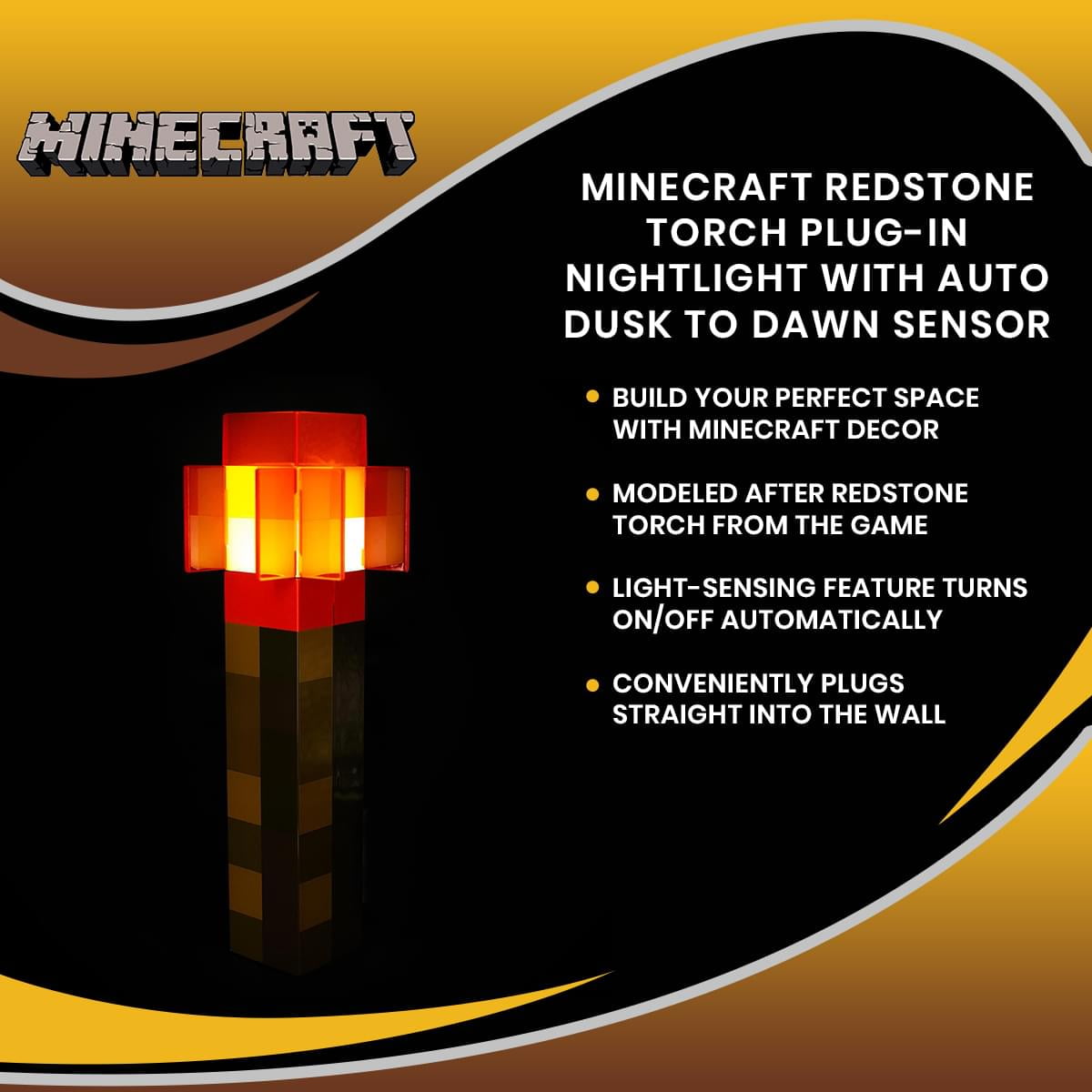This image showcases a detailed advertisement for a Minecraft-themed product. The background features a striking yellow and black color scheme. Prominently displayed in white letters, the top section announces "Minecraft" alongside the product name: "Minecraft Redstone Torch Plug-In Nightlight with Auto Dusk to Dawn Sensor." Below the main text, four bullet points provide additional information: "Build your perfect space with Minecraft decor," "Modeled after Redstone Torch from the game," "Light sensing feature turns on/off automatically," and "Conveniently plugs straight into the wall." On the left side of the image, extending from the middle to the bottom, there's an illustration of the Redstone Torch nightlight, showcasing a design reminiscent of the iconic torch from the game, complete with a red lit top and a brown handle. The text and graphics are enclosed in a curved, gold border that enhances its visual appeal, making it a captivating piece of Minecraft-themed decor.